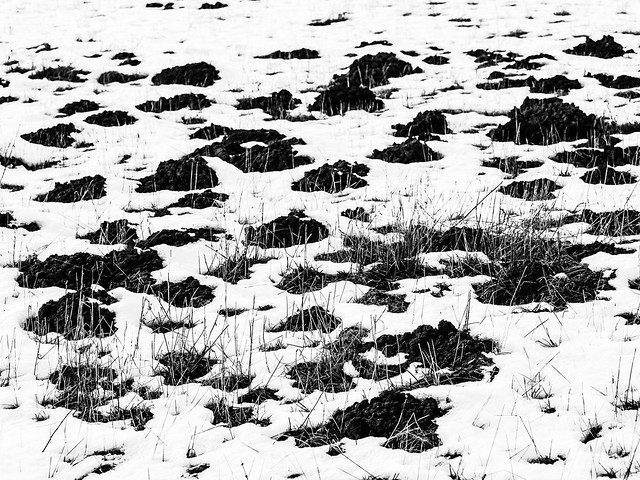This black and white photograph captures a desolate, snow-covered field in winter. The image is taken from the perspective of someone standing on the ground, looking into the distance. Scattered across the snowy expanse are numerous dark patches that seem to be either dirt, rocks, or possibly grass, with small twigs or weeds poking through. These dark mounds create the appearance of islands in a white sea. As the eye travels further back in the photo, the density of these black patches appears to thin out. The stark contrast between the snow and these black elements gives the scene a monochromatic and textured appearance, contributing to its bleak yet intriguing landscape.